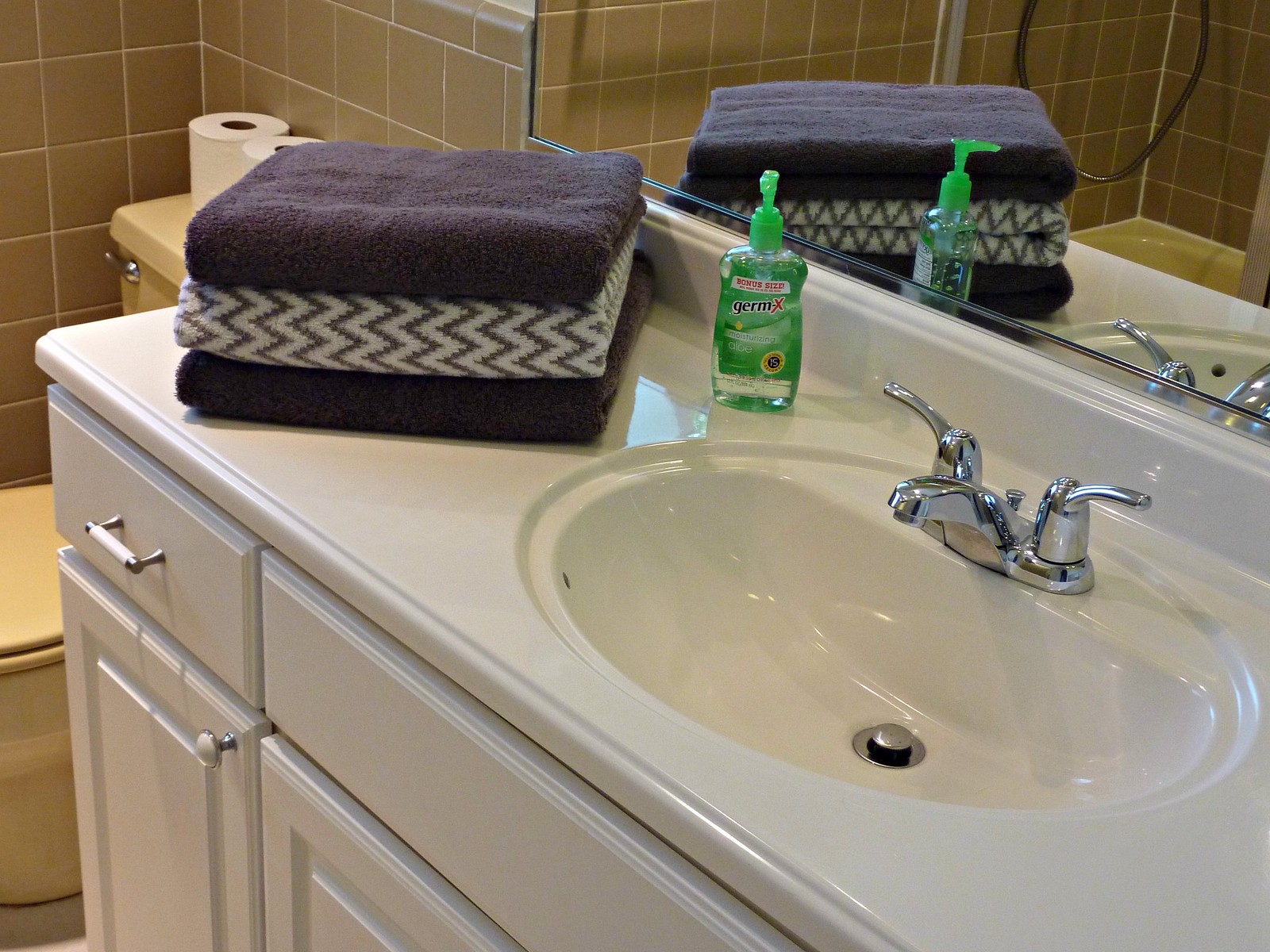The image showcases a pristine bathroom sink set within a white vanity. Adorning the vanity are three neatly stacked towels: a blue towel at the bottom, a white towel with blue stripes in the middle, and another blue towel on top. The sink features a two-handle silver faucet, gleaming against the white counter. Additionally, the vanity has a visible drawer, its handle crafted from silver with a white center, complemented by a matching knob below. To the right of the towels but left of the sink sits a soap bar labeled "Euromax." In the background, an almond-colored commode is situated in the corner, bordered by brownish tiles that accentuate the overall decor. Also visible in the image is a mirror reflecting parts of the bathroom, completing this detailed glimpse into the well-kept space.